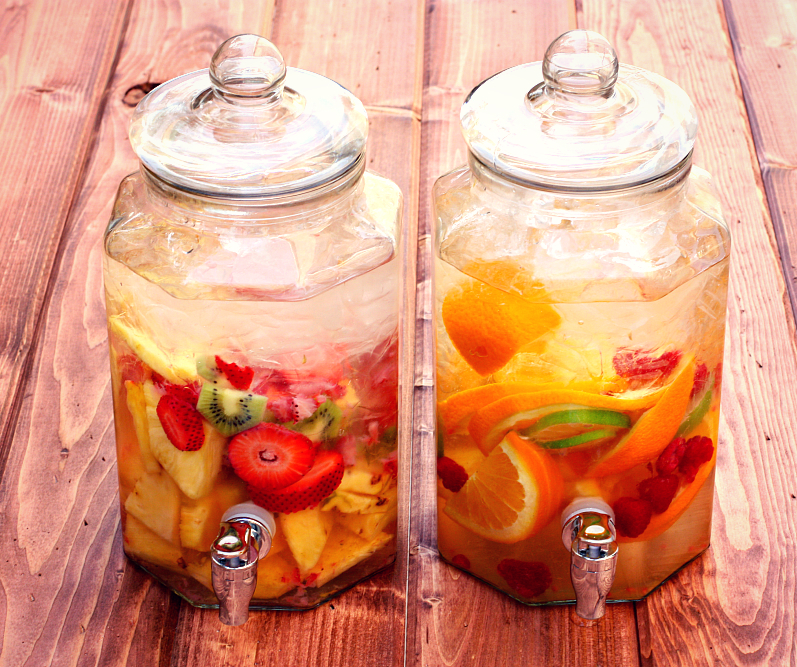This image captures two glass jars set on a wooden table, reminiscent of a picnic setting, with intricately detailed swirls of wood grain visible on the planks. Each jar is equipped with a spout for convenient pouring. The left jar contains an enticing mix of sliced strawberries, kiwis, and what looks like pineapple, all submerged in water with ice, suggesting a refreshing fruit-infused beverage. The right jar is filled with a colorful blend of oranges, limes, raspberries, and possibly lemon, similarly submerged in ice water. Together, these aesthetically pleasing and mouth-watering jars of fruit-infused water form an inviting and perfect centerpiece for a leisurely and refreshing summer picnic.